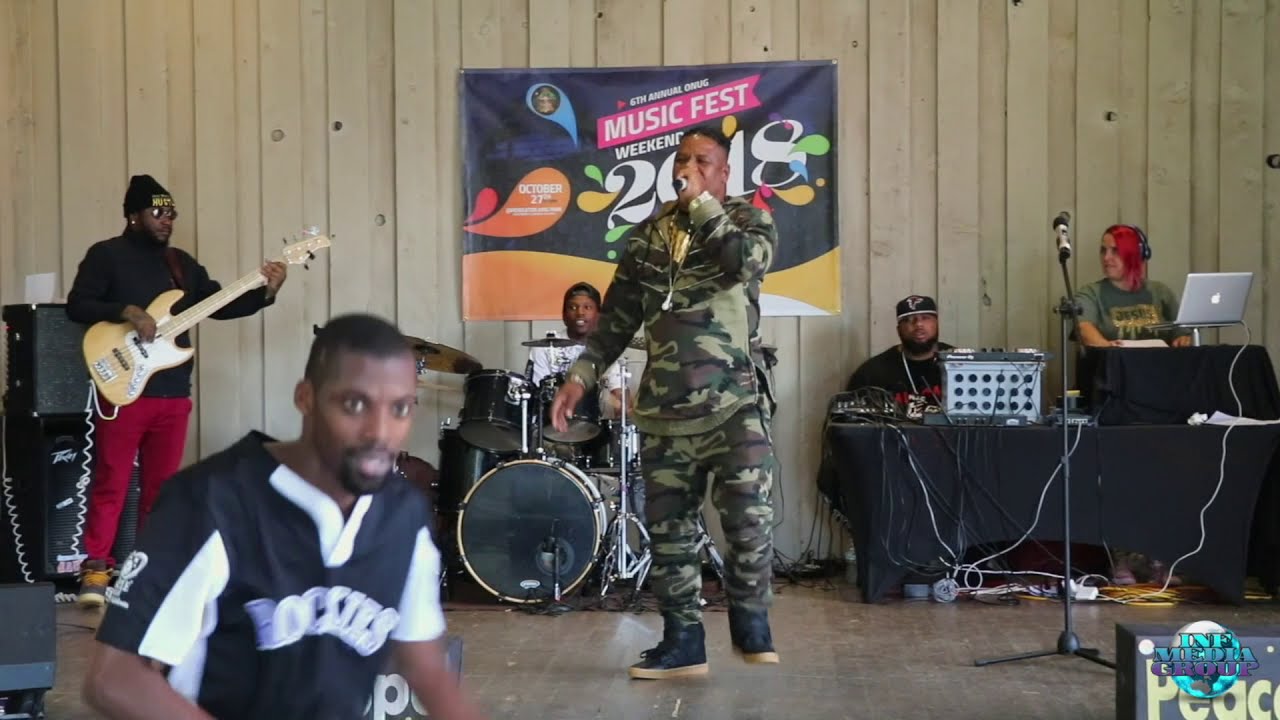In the image, a band is performing indoors on a hardwood floor. Central to the image is an African American male in a military outfit, featuring green camo pants and a green camo sweater, complemented by black boots with gum soles. He wears gold chains and has short black hair. He holds a microphone close to his face, indicating he is singing.

To his left, a male bass guitarist with long dreads and a black beanie is playing a light wood-colored bass guitar. He wears a black jacket and red burgundy pants. In the background, another African American male drummer with a backwards black hat and a white shirt plays on a black drum kit.

Positioned to the right is a black male sitting at a table with mixer controls, likely handling the audio work. Next to him, a white woman with red hair and headphones is focused on a Mac laptop, possibly monitoring the sound.

A poster in the backdrop reads "Music Fest Weekend 2018," tying the scene together as a music festival event. The image is rich with color, including light brown, black, red, green, light blue, and orange. Despite the festival theme on the poster, the setting appears to be an indoor practice session rather than an outdoor fest.